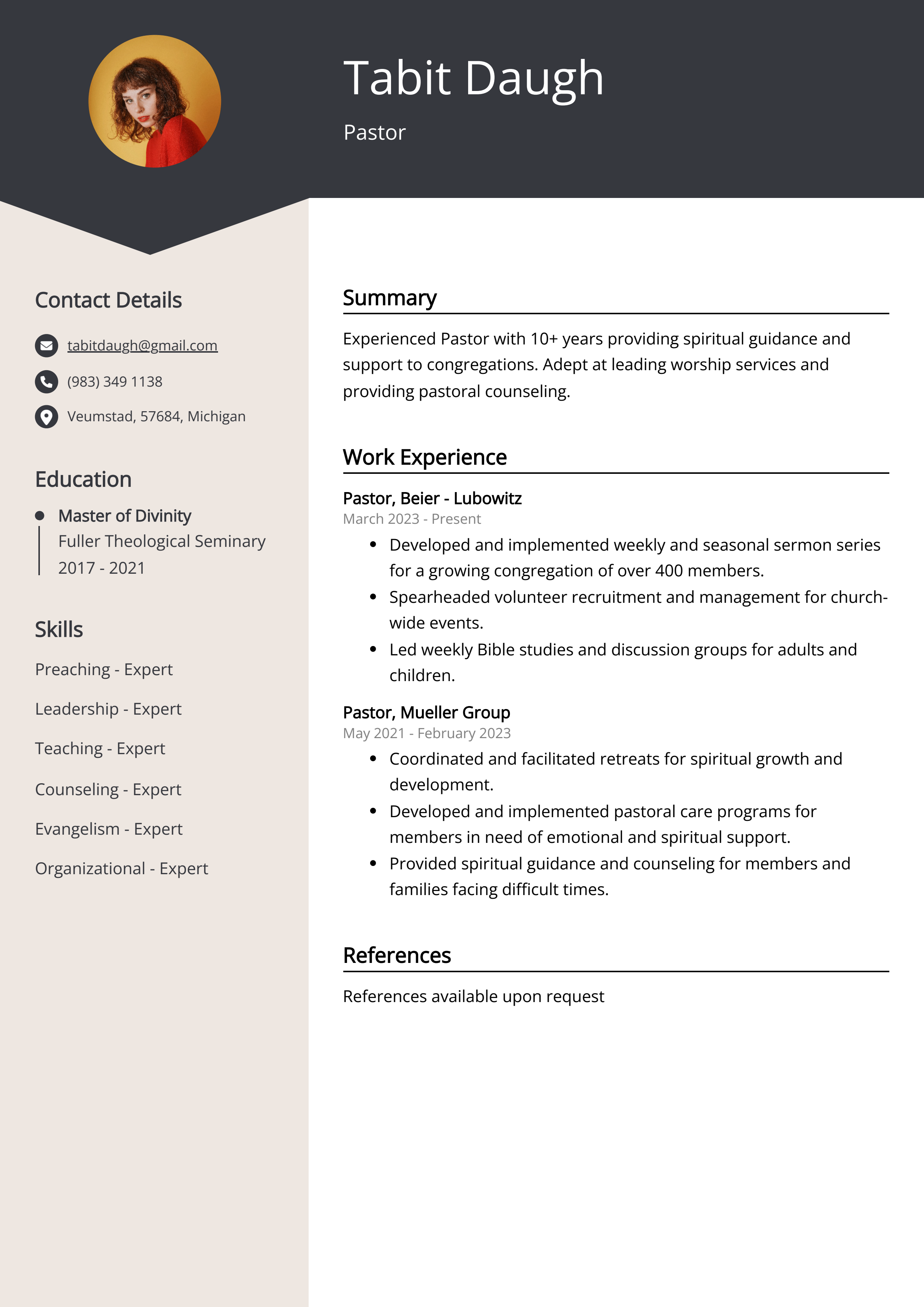This vertically-aligned resume portrait features a prominently black header at the top, highlighted by a pristine white inscription of the name "Tabitha Daugh" and the designation "Pastor." Centrally positioned within this black border is a circular headshot of a young woman, Tabitha, sporting short curly brown hair, red lips, and a vibrant red shirt, posed against a yellow background.

Directly beneath this header, the resume divides into two columns. The left column, shaded in a light gray or beige tone, systematically organizes her contact details, education, and skills. This section begins with icons denoting her email, phone number, and location details. Following these, her academic credentials are listed, spotlighting a Master of Divinity from Fuller Theological Seminary, completed between 2017 and 2021.

In contrast, the right column retains a white backdrop and elaborates on her professional narrative. This section starts with a "Summary" header, underlined for emphasis, followed by a comprehensive paragraph detailing her pastoral experience. Beneath this, "Work Experience" is outlined, showcasing her employment history with multiple organizations in pastoral roles. Finally, the resume concludes with a "References" section, also underlined, stating "References available upon request" at the bottom.